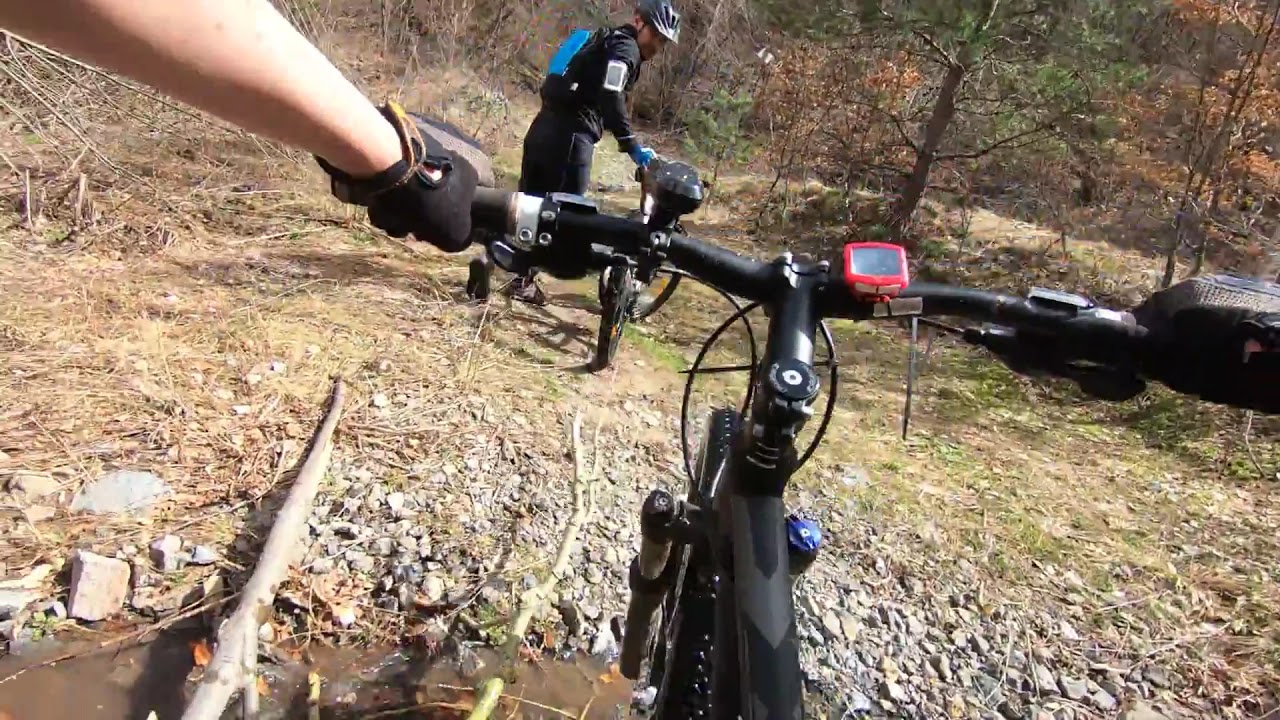This detailed photograph, captured from the chest perspective of a GoPro, offers an immersive view of a mountain biking experience. The viewer's vantage point is low on a black bike equipped with a red mileage counter and a prominent front light. The handlebar occupies the center of the image, with a white hand clad in a black glove gripping it from the top left. The path ahead includes a small creek with surrounding rocks and scattered mud patches, indicating the crossing of a watery, rugged terrain. This area, with sparse grass and numerous dead tree branches, suggests a setting in early spring or late fall when foliage has yet to flourish.

The scene is part of a forest trail, lined with sporadic, leafless trees. Ahead, another biker, a white male in a black helmet and long-sleeved fitness outfit, turns to face the camera while pushing his bike. This biker also wears a backpack and stands amidst the trail, emphasizing the challenging nature of the descent. The image encapsulates the adventurous spirit of mountain biking through tough, natural terrain.